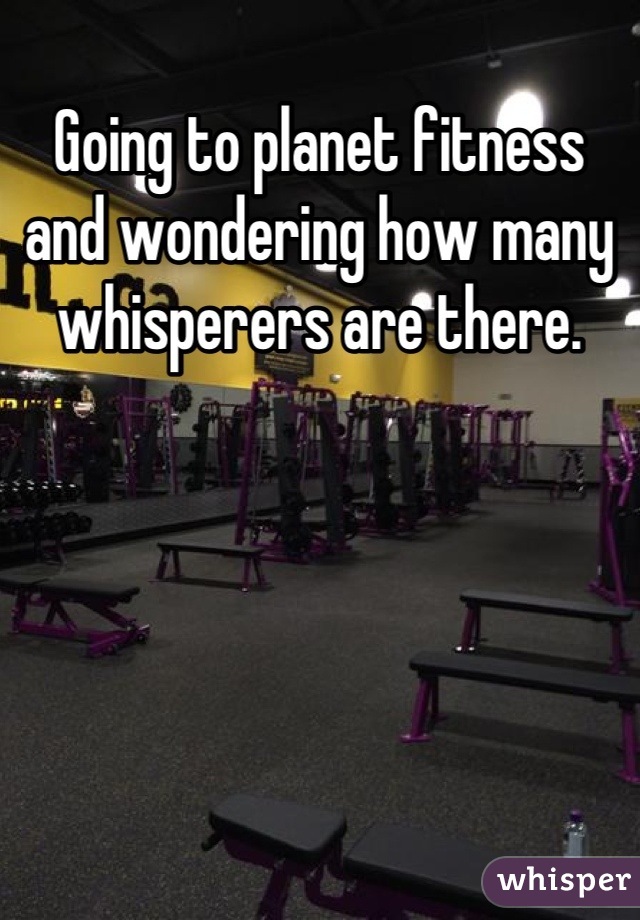The image captures a dimly lit, empty Planet Fitness gym. The setting is primarily dark, with a spotlight or bright light hanging from the ceiling. The text, "Going to Planet Fitness and wondering how many whisperers are there," is displayed prominently in large white letters across the upper part of the image. The gym is equipped with various pieces of weightlifting equipment, mostly black, with some benches featuring red or purplish-pink accents. The floor appears to be black or dark gray, and there's a water bottle in the lower right-hand corner with the word "Whisper" beneath it. A long mirrored wall stretches across one side of the gym, reflecting some dumbbells and more equipment. Above this mirrored wall, there is a long yellow section possibly featuring Planet Fitness's logo and lettering.